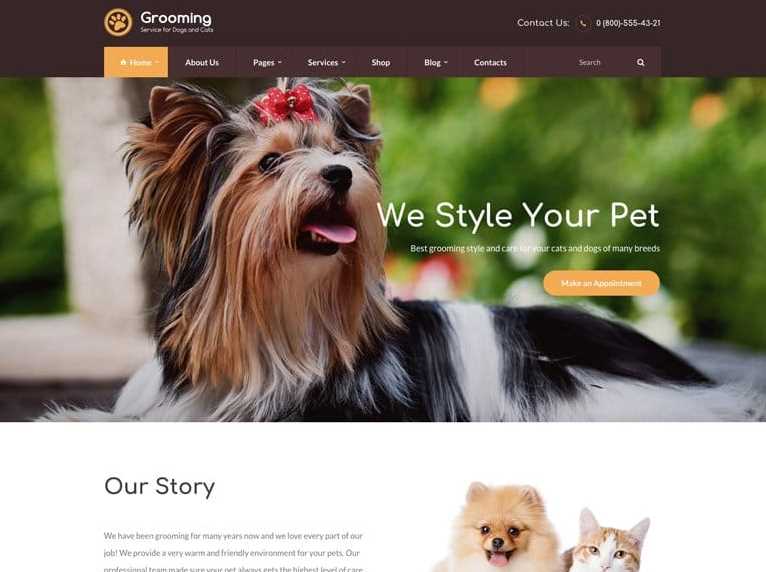This image features a horizontally oriented screenshot showcasing a beautifully groomed Yorkie dog, captured in a profile view of its left side. The Yorkie, adorned with a red bow on the top of its head, strikes a charming pose with its face pointed forward. To the right of the Yorkie, bold white text states "We style your pet," accompanied by a yellow action button that reads "Make an appointment."

In the upper left corner, the name of the website, "Grooming Service for Dogs and Cats," is displayed against a black header, featuring a yellow paw icon encircled in yellow. Below the image of the Yorkie, the text "Our Story" is visible, while to the right, there is a colorful photograph of a Pomeranian and an orange tabby cat, contributing to the appealing visual design of the page.